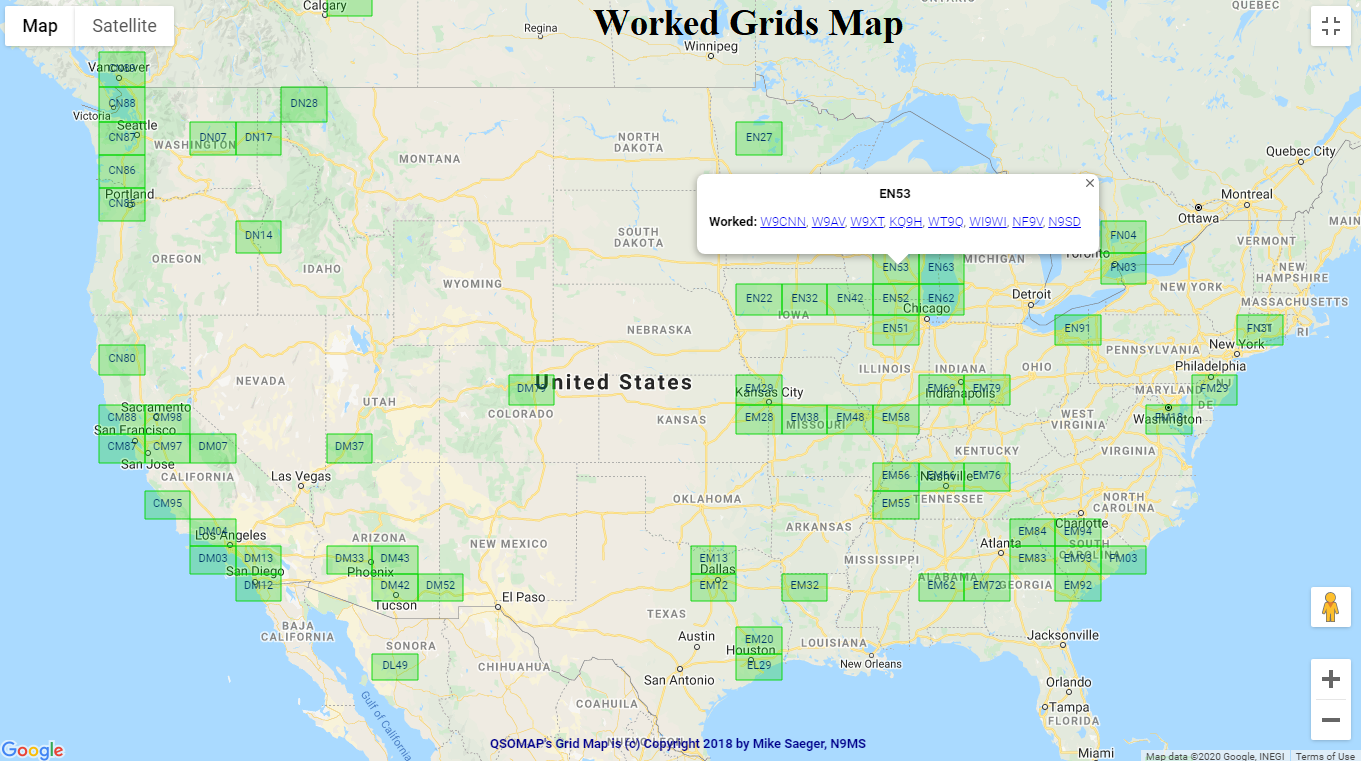A detailed caption for the given image could be:

"An intricately detailed map titled 'Worked Grids Map' in bold black text dominates the top. Centered on the United States, the map's base is shaded in gray to represent land, while bodies of water are depicted in light blue. The map clearly displays the outlines of all 50 states. Scattered across this map are green squares, some isolated and others grouped in pairs or trios.

At the top of the map, within a white rectangular banner, the label 'EN 53 worked' is highlighted alongside seven blue tabs. The map interface includes various functional icons: 'map' and 'satellite' in the top-left corner, a maximize icon in the top-right corner, and zoom controls (plus and minus symbols) in the bottom-right corner. Additionally, a blue copyright notice stretches across the bottom, adjacent to a small Google logo located in the bottom-left corner."